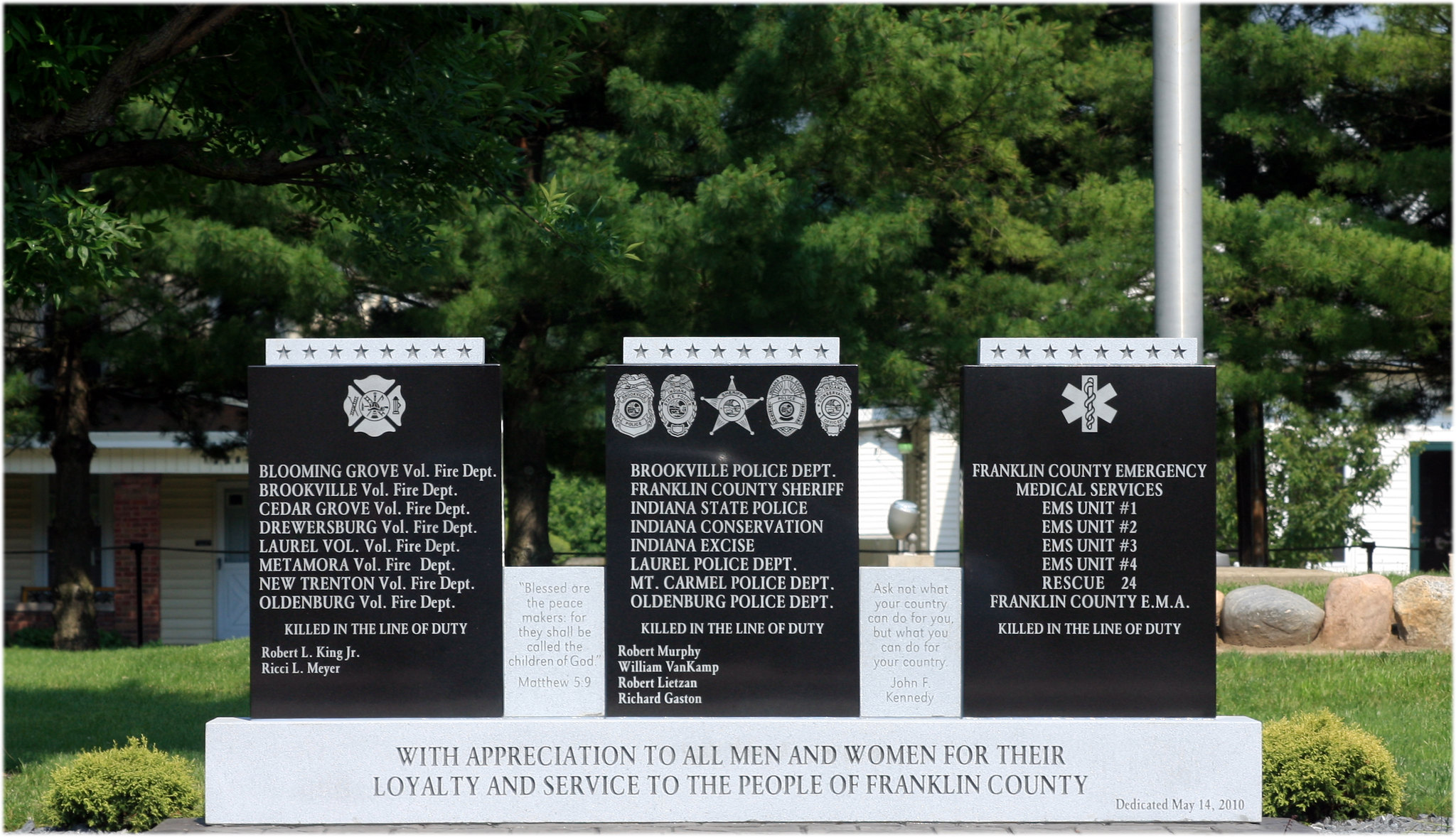In the outdoor photo, three prominent black stone memorials are situated in a landscaped garden, bathed in sunlight. Each memorial features distinct inscriptions and symbols to honor different public service divisions. 

On the leftmost black stone, eight stars are etched across the top, and at the summit, a badge is carved. The inscription reads: "Blooming Grove Vol. Fire Department, Brookville Vol. Fire Department, Cedar Grove Vol. Fire Department, Jewisburg Vol. Fire Department, Laurel Vol. Fire Department, Metamora Vol. Fire Department, New Trenton Vol. Fire Department, Oldenburg Vol. Fire Department," followed by "Killed in the Line of Duty: Robert L. King Jr., Rizzi L. Meyer." Below this, situated between the left and center memorials, a small grey stone bears the biblical inscription: "Blessed are the peacemakers, for they shall be called the children of God. Matthew 5:9."

The central stone displays five badges aligned at the top, with a prominent five-pointed star at the center. The engraved text lists: "Brookville Police Department, Franklin County Sheriff, Indiana State Police, Indiana Conservation, Indiana Excise, Laurel Police Department, Mount Carmel Police Department, Oldenburg Police Department," and commemorates "Killed in the Line of Duty: Robert Murphy, William Van Kamp, Robert Leitron, Richard Gaston." Adjacent to this plaque, a small grey stone bears a quote from John F. Kennedy: "Ask not what your country can do for you, but what you can do for your country."

The rightmost memorial features an asterisk and an emblem of a snake encircling a pole, topped with eight stars. The grey text honors: "Franklin County Emergency Medical Services, EMS Unit 1, EMS Unit 2, EMS Unit 3, EMS Unit 4, Rescue 24, Franklin County EMA, Killed in the Line of Duty." 

The three black stone memorials are mounted on a shared grey stone base, which is inscribed with a dedication: "With appreciation to all men and women for their loyalty and service to the people of Franklin County. Dedicated May 14, 2010." The photo also captures green grass, trees, and rocks in the background, adding to the serene and reverent atmosphere of the scene. A yellow house with a red brick wall stands to the left, and another white house with blue trim is visible to the right, both amidst the greenery. Black poles with chains and well-kept bushes flank the statues, further contributing to the tranquil setting.